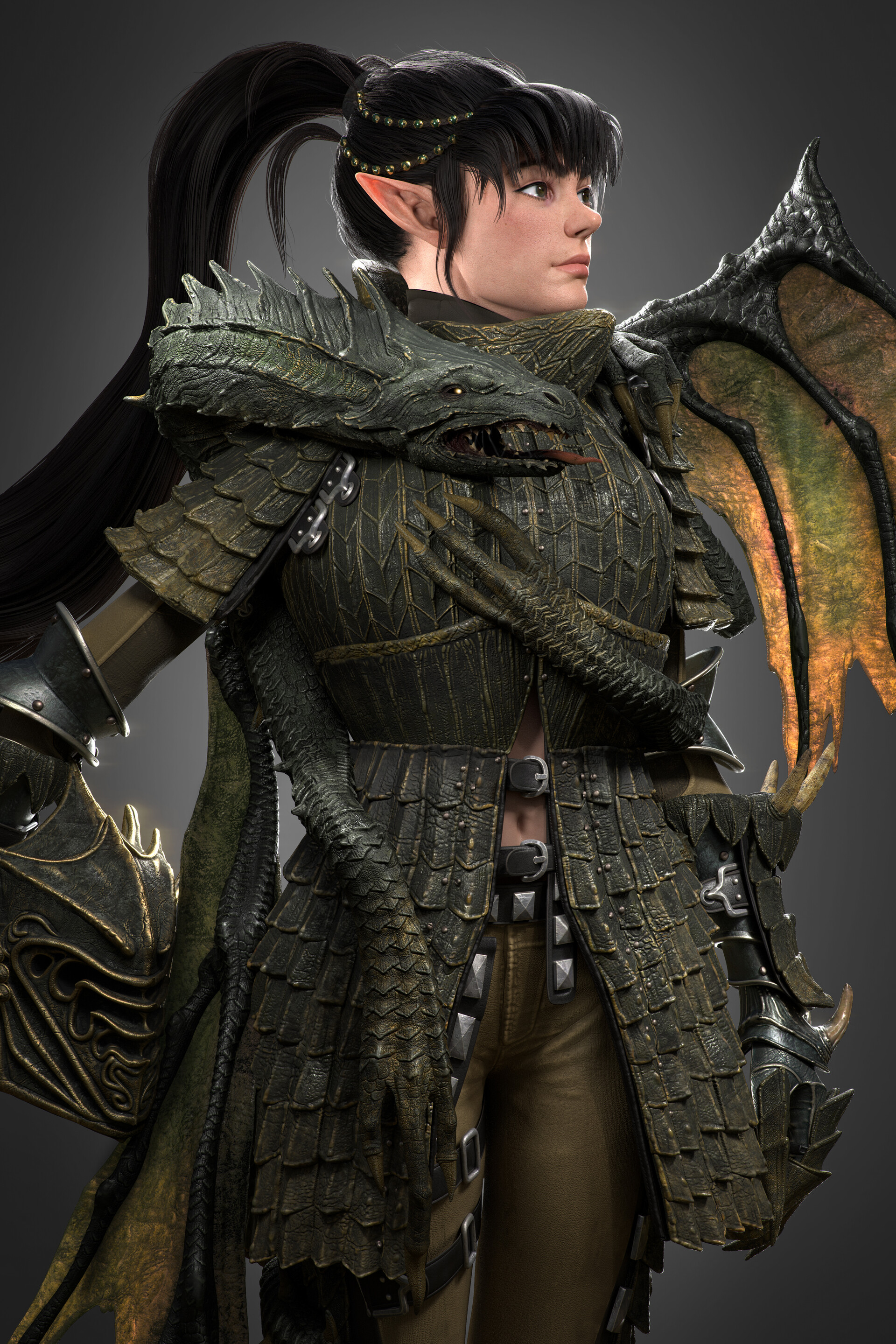In this detailed 3D-rendered image, we see a full-color, vertically rectangular depiction of a Caucasian female elf warrior, positioned against a predominantly black background that subtly illuminates around her, offering a gradient effect. She stands in a side view, gazing off to the right. Her thick black hair is tied back into a ponytail, accentuating her pronounced elf ears. The elf is clad in elaborate, dark green armor crafted from leather, which exudes a fantastical essence. The armor is adorned with intricate dragon-themed details: a dragon head and wing embellish the shoulders, and draconic claws and heads are scattered across the jacket and shoulder pads. Her armor extends down just below her hips, flaring slightly at the sides, and is paired with olive green pants. Resting on her shoulders and draping along the sides is a dragon, with its head visible on one side and its wing on the other, adding to the majestic and formidable appearance. Completing her ensemble, she holds a dark green helmet, outlined with golden lines, in her left hand. The background adds to the mystical ambiance, shifting from black to a subtle gray around the figure.